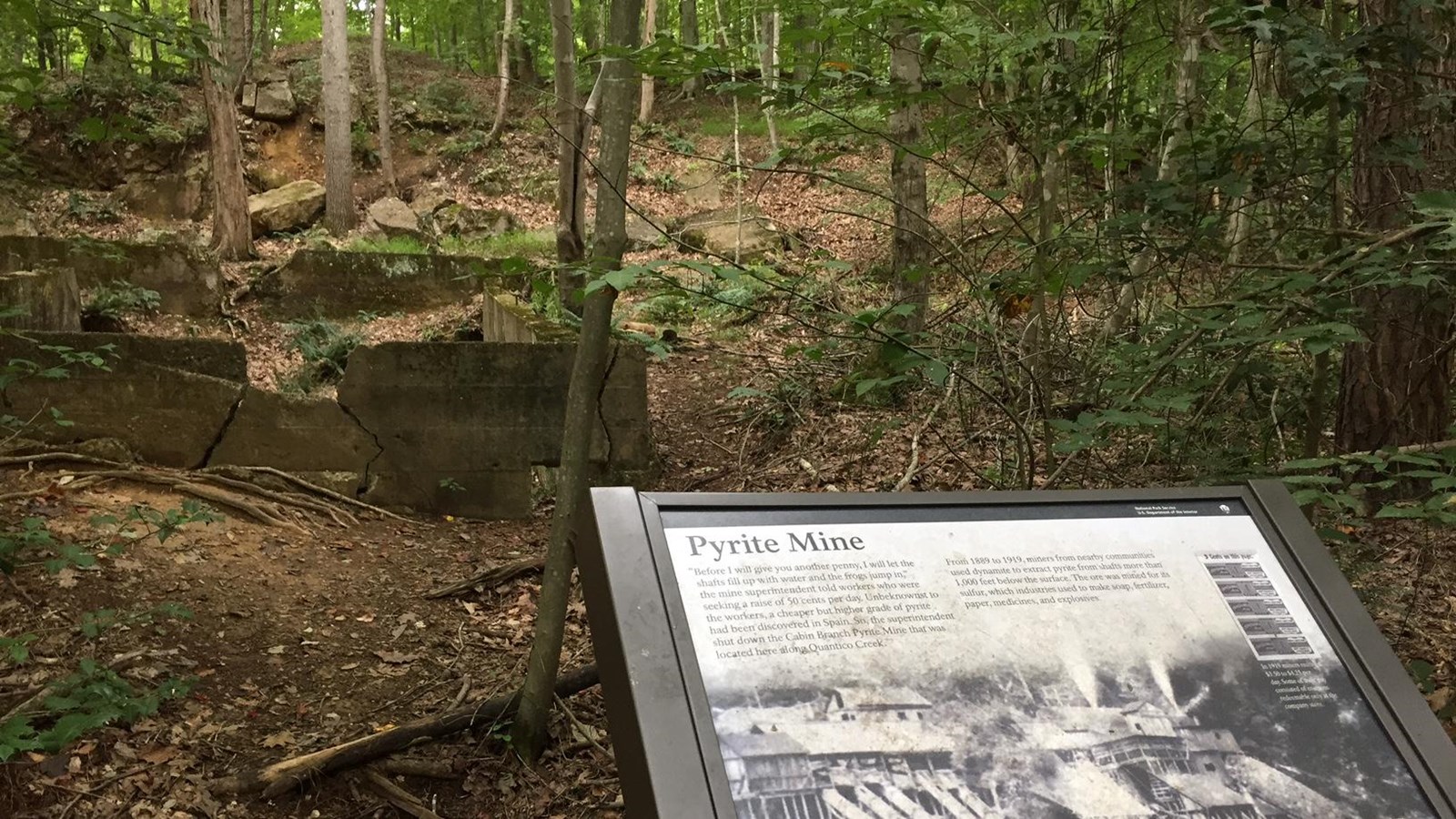The photograph depicts a forested setting with many thin, skinny trees and a forest floor covered in fallen leaves. Prominently featured in the foreground is an informational kiosk bearing a large black and white image and the heading "Pyrite Mine." The sign includes text detailing the history and significance of the old mine, though much of the text is too small to be legible. The black and white photo on the sign shows what the expansive mining area used to look like, with historical buildings faintly visible. Adjacent to the sign, the remnants of a dilapidated brick and concrete wall can be seen, which appear cracked and broken down, blending into the natural surroundings. The scene is devoid of any active pathways, conveying a sense of abandonment and reclamation by nature.